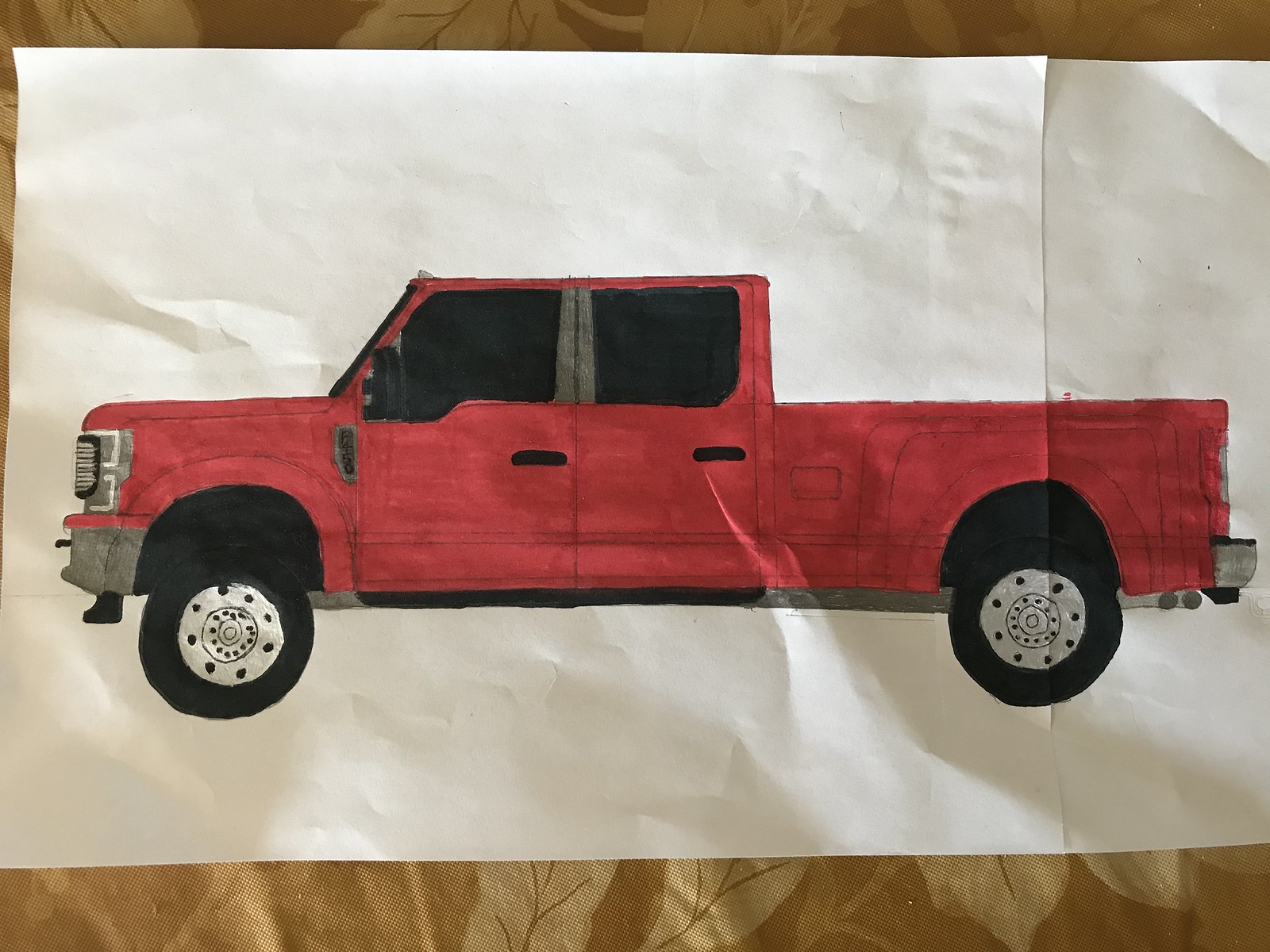A meticulously drawn red pickup truck dominates this artwork, which spans across two conjoined sheets of white paper. The vibrant red truck features black-tinted windows, silver or chrome bumpers, and hubcaps, along with black wheels, suggesting a modern design. The truck is the sole subject of the drawing, which is set against an unadorned white background. The sheets of paper, slightly wrinkled and curling at the edges, rest on a luxurious gold tablecloth adorned with a pale gold floral pattern. The vehicle appears to be vividly colored, possibly using paint or markers, rather than crayons, giving it a rich and uniform texture.